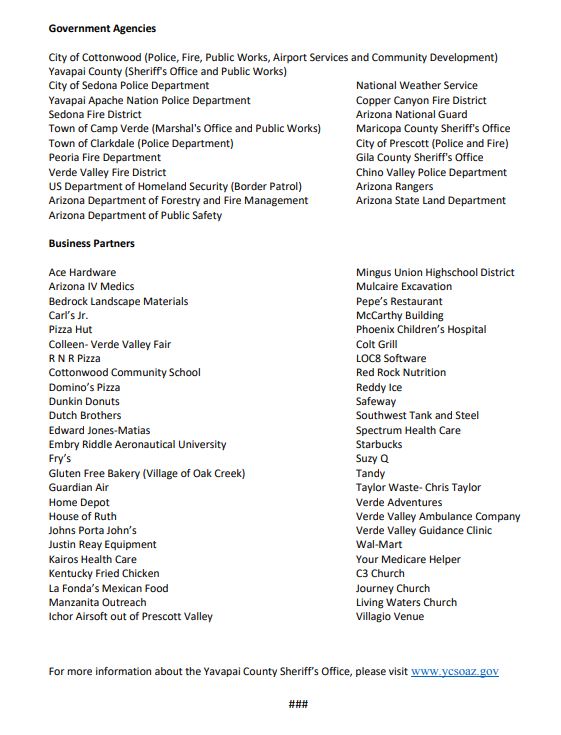This image features a detailed screenshot of two comprehensive lists: government agencies and business partners. At the top left, the title "Government Agencies" is prominently displayed in bold black font. Below this title, an extensive list of various agencies is enumerated, including:

- City of Cottonwood
- Yavapai County
- City of Sedona Police Department
- Yavapai-Apache Nation Police Department
- Town of Camp Verde
- Town of Clarkdale
- Paria Fire Department
- Verde Valley Fire District
- U.S. Department of Homeland Security Border Control
- Arizona Department of Forestry and Fire Management
- Arizona Department of Public Safety
- National Weather Service
- Copper Canyon Fire District
- Arizona National Guard
- City of Prescott
- Yavapai County Sheriff's Office
- Chino Valley Police Department
- Arizona Rangers
- Arizona State Land Department

Beneath this section is another list labeled as business partners, featuring well-known establishments such as:

- Carl's Jr.
- Pizza Hut
- Safeway
- Susie Q
- Guardian Air
- Home Depot
- House of Ruth
- Walmart

These lists highlight both the government and business entities collaborating with the organization. At the very bottom of the document, additional information about the Yavapai County Sheriff's Office is provided, along with a hyperlink to their website, www.ycsoaz.gov, displayed in blue text indicating it is clickable for more information.